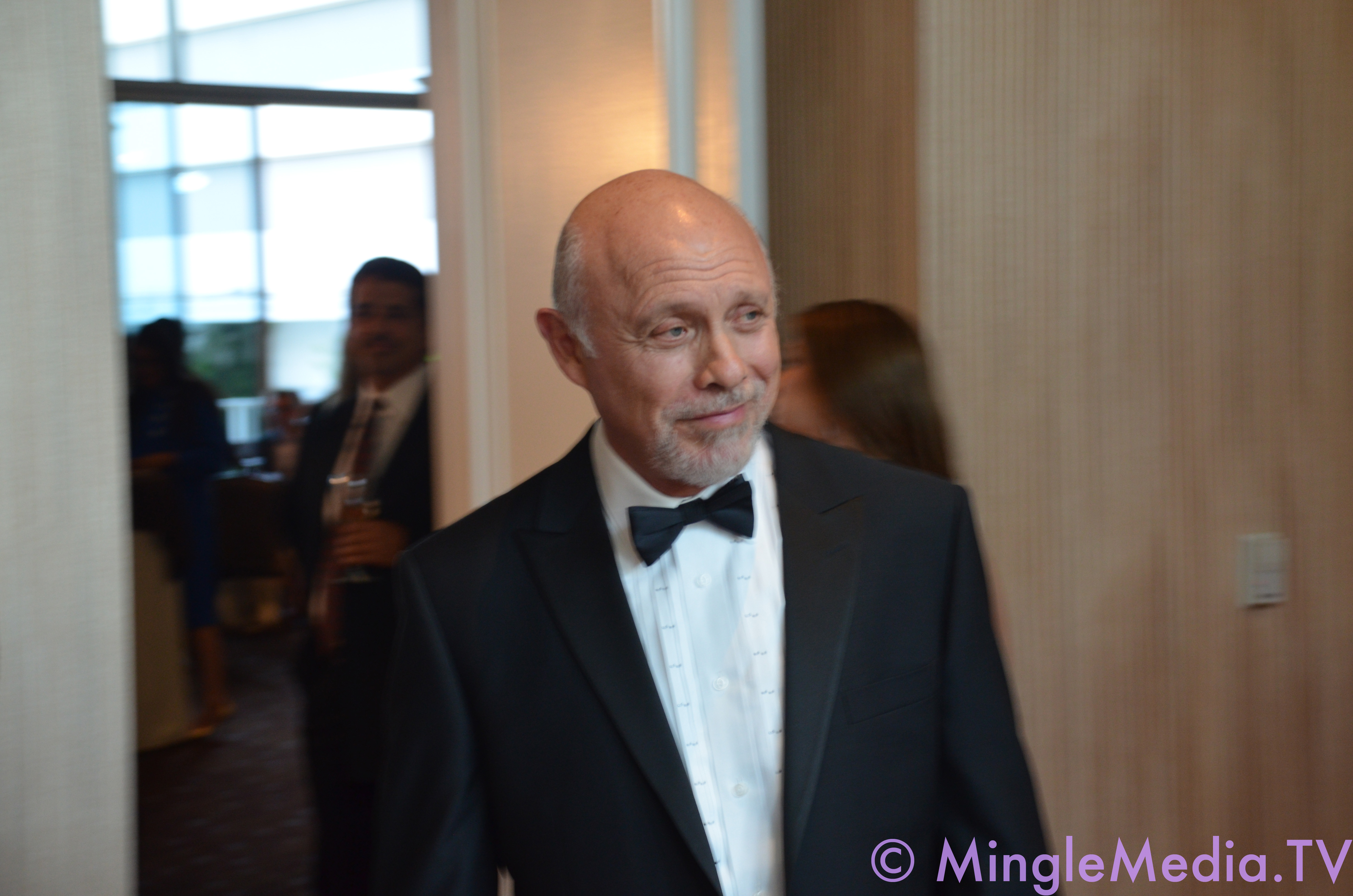The photograph features the actor Hector Elizondo, who is well-known for his roles in The Princess Diaries movies and Grey's Anatomy, typically portraying father-figure characters. In this vibrant, color image, he is dressed formally in a black tuxedo with a white button-down shirt and a black bow tie, exuding a sophisticated demeanor. Hector Elizondo stands confidently, his gaze slightly directed to his left with a subtle smile on his face. He is bald on the top, with gray hair on the sides, complemented by a matching gray mustache, beard, and goatee. The background shows a slightly blurred ambiance of an elegant setting, presumably the entrance to a ballroom or similar venue. People dressed in formal attire, including a man with a drink and a woman walking past, add to the scene's lively atmosphere. A wooden-colored wall with a light switch is visible, and the bottom right corner of the image displays the watermark "Mingle Media TV," indicating the source. The natural lighting in the photograph enhances the clarity and vividness of the moment captured.